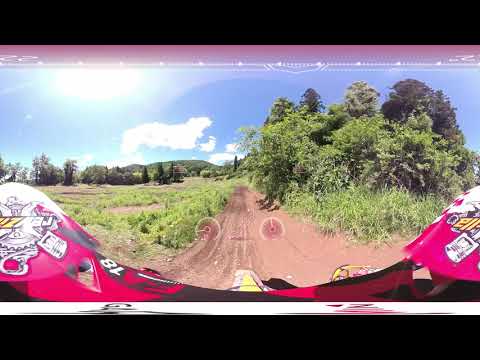In this vibrant 360-degree image taken from the perspective of a vehicle, we look through a windshield bordered top and bottom by solid black rectangles framing the scene. The dashboard, likely belonging to a racing motorcycle or sporty vehicle, features two small, round dials and a red panel adorned with various stickers and numbers. Ahead, a long, brown dirt road stretches into the distance, flanked by patches of green grass and areas where the ground is bare. On the right, a variety of tall, bushy green trees line the road, while the left side is more open, with fewer trees but a soft green backdrop. A low hill rises on the horizon, beneath a bright blue sky dotted with fluffy white clouds. The sun shines brightly, its glare noticeable on the left side of the image. The setting is indicative of the outdoors, in the middle of the day, capturing the essence of a dirt biking path.